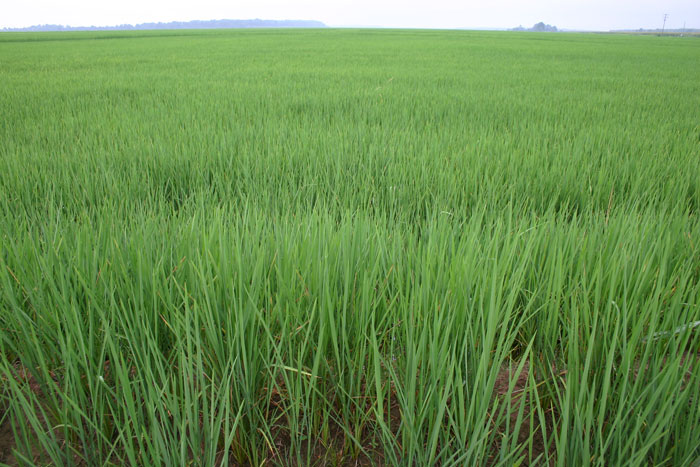The outdoor photograph showcases a vast, green grassy field extending from the foreground to the distant background. The majority of the picture is dominated by this lush greenery, with visible patches of brown soil at the base, suggesting a potential crop or grass that has yet to fully develop. In the distance, there are mountain ranges that span from the top middle to the corners of the image, capped by a mix of white and blue sky. On the right side, there are some trees and blurred structures that might be buildings or potentially a small town, adding depth to the scene. The color palette of the image includes vibrant greens, earthy browns, light neutral tones, and hints of bluish hues in the sky, capturing the essence of a serene, expansive landscape in the grassy plains.